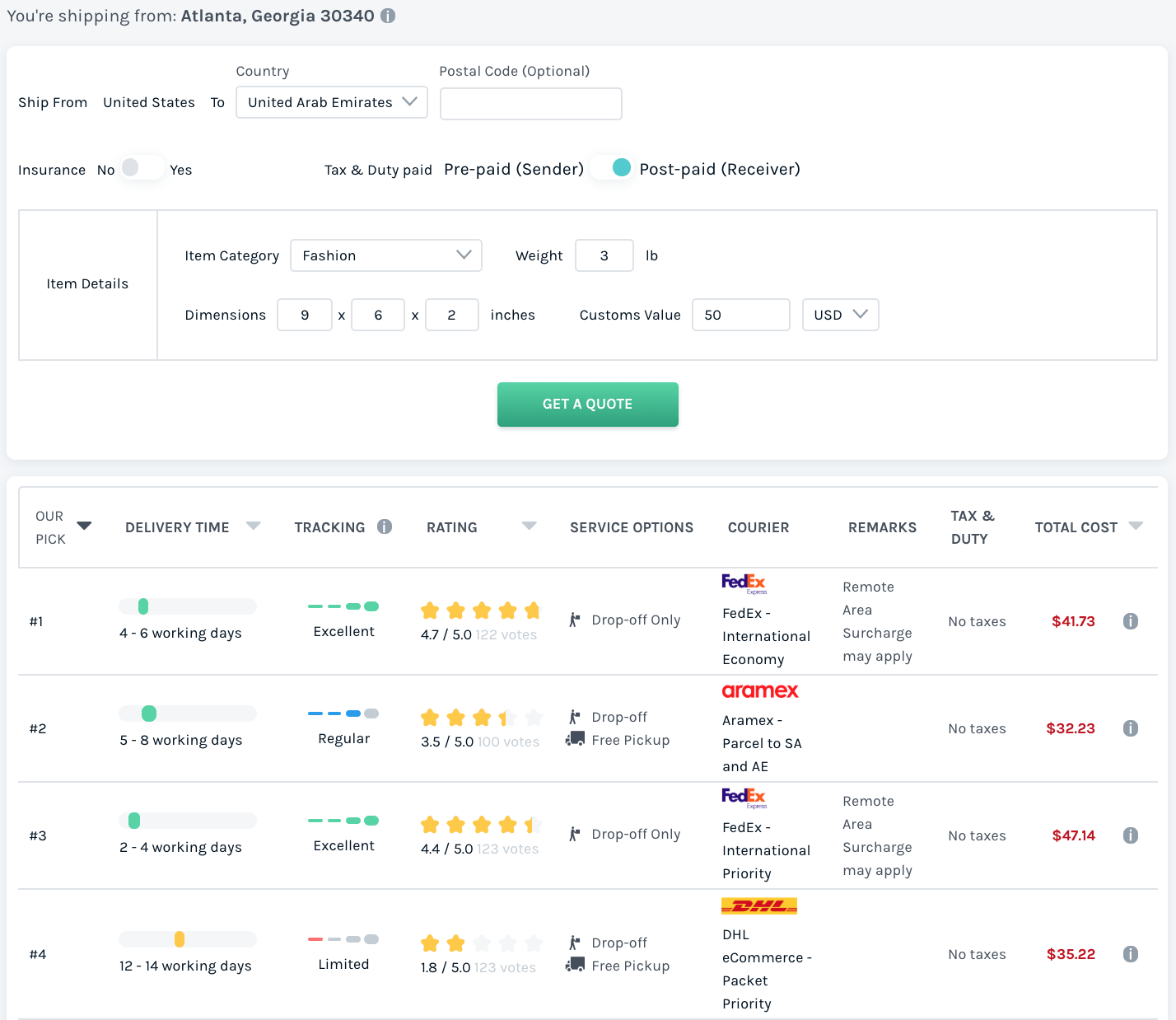The image depicts a detailed section of a shipping website interface. At the very top left, the shipping origin is specified as "Atlanta, Georgia 30340." Directly below, it reads "Ship from United States to" with a drop-down menu for selecting the destination country; the selected country is displayed as "United Arab Emirates." An optional postal code field follows beneath.

Further down, there's a section for insurance options, labeled as "Insurance," with choices for "Yes" or "No." Adjacent to this is some text reading "Tax and Duty" with options for "Prepaid (Sender)" indicated by a small green button, and "Post Paid (Receiver)."

The next segment is titled "Item Details," which includes fields for the item's category, weight, dimensions, and customs value. The selected item category from the drop-down menu is "Fashion," with the weight listed as "3 pounds." The dimensions are noted as "9 by 6 by 2 inches," and the customs value is "$50 USD."

Below this information, there's a prominent green button with white text labeled "Get a Quote."

The bottom section presents various shipping options, each specifying the carrier, estimated working days for delivery, and respective costs. The carriers listed include two options for "FedEx," one for "Aramex," and one for "DHL." Each option displays the price on the right-hand side and the estimated working days to the left.